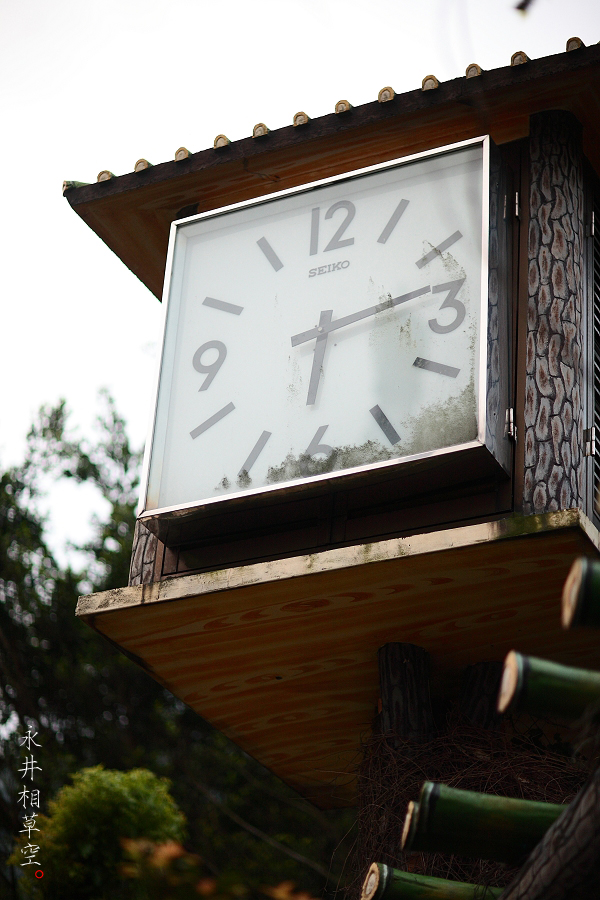This outdoor photograph captures a square clock mounted on a dark wooden structure. The clock features a minimalist white background with black hour markers in the form of ticks, and bold black numbers at 12, 3, 6, and 9 o'clock positions. The black hour and minute hands stand out clearly against the light face. In the bottom left corner, there is Japanese writing in white. Green piping runs along the roof of the house and is also visible in the bottom right corner. Lush green trees form a serene backdrop, adding a natural contrast to the crafted elements in the foreground.